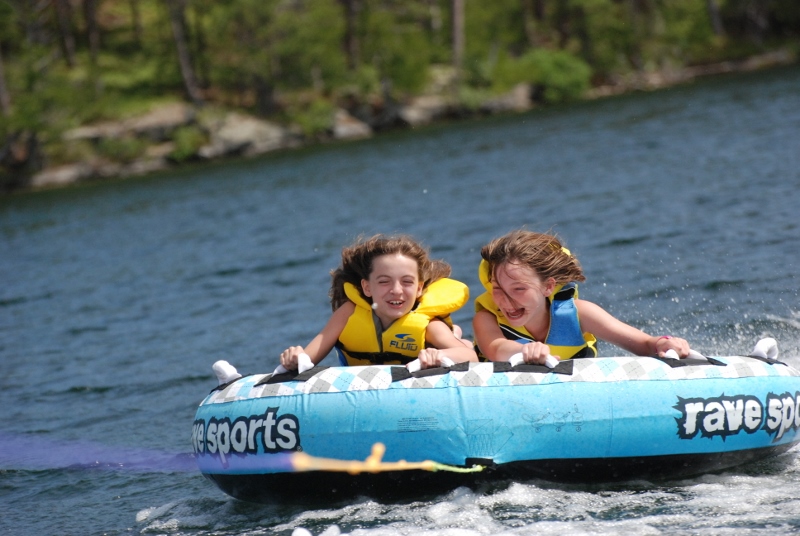This vibrant daytime photograph captures two young children, most likely between 6 and 9 years old, having an exhilarating time on a large, inflatable river raft. The raft, marked with the white lettering "Rave Sports," is round and equipped with multiple white handles for secure gripping. The children, both with brown hair fluttering in the breeze, are firmly holding onto the handles. The child on the left sports a yellow life preserver vest, while the one on the right wears a yellow and blue life preserver vest. Their raft appears to be moving swiftly across a large, relatively calm body of water, which stretches out to a distant, blurry shoreline. This shoreline is adorned with a mix of greenery, including trees, underbrush, and climbable rocks. The bright daylight ensures every detail is vividly captured, showcasing the playful and adventurous spirit of the moment.